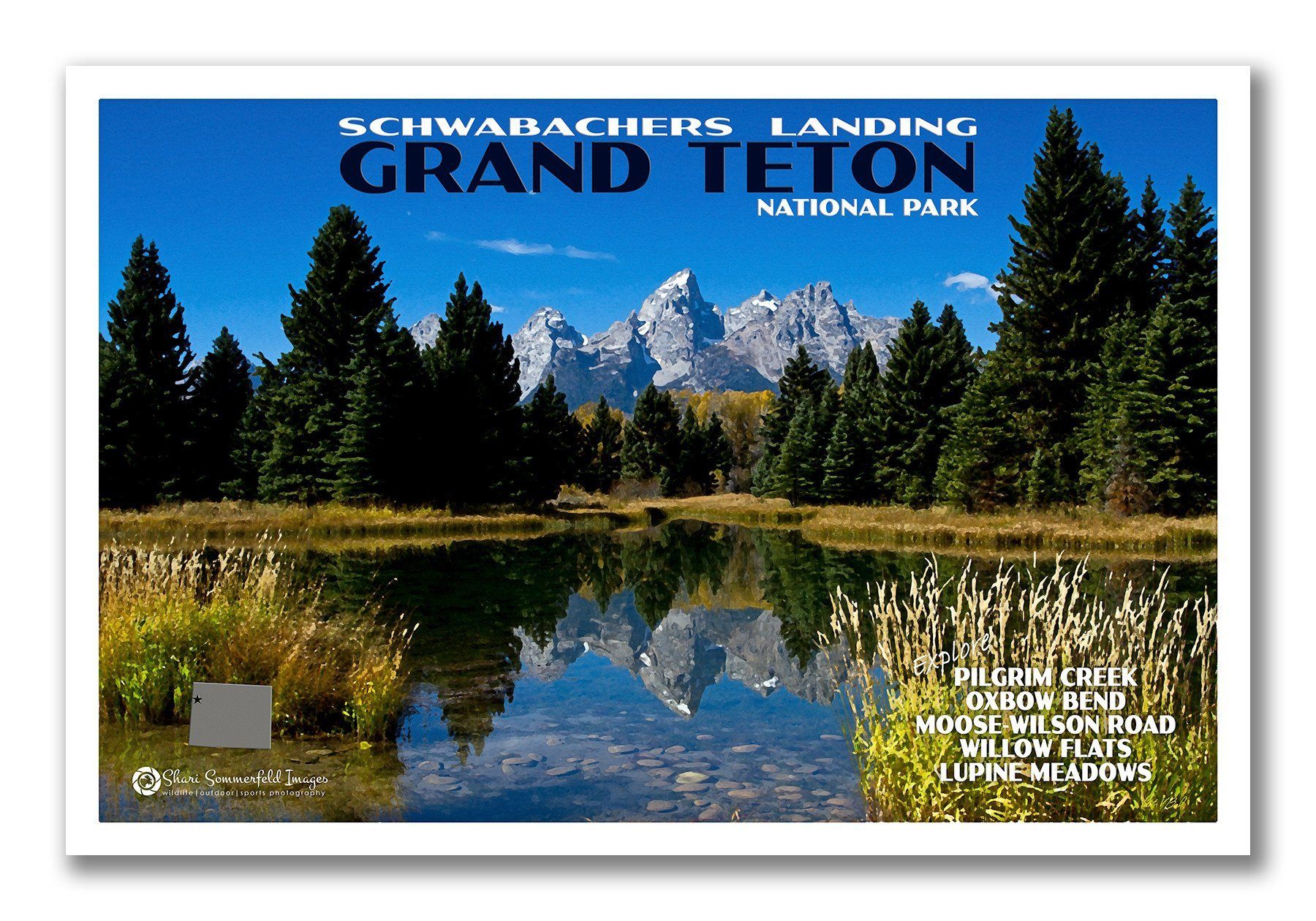This highly detailed travel poster for Schwabacher's Landing in Grand Teton National Park portrays a stunning, photographic-like painting of a serene mountain scene. Dominated by the dark gray, snow-capped peaks of the Teton Mountains in the center, the composition reflects the majesty of nature against a backdrop of a vibrant blue sky decorated with wispy white clouds. Flanking the mountains are dense, dark green to black pine trees, which, along with their reflections, frame the tranquil lake occupying the bottom half of the image. 

Golden tufts of grass mixed with hints of green enhance the landscape, while clusters of brown sprigs and rounded, beige stones adorn the lake's edge. The perfect mirror image of the mountains and trees in the lake adds a mesmerizing symmetry to the scene. The bottom left corner features the logo of Sherry Sommerfeld Images Wildlife Outdoor Sports Photography, with the corresponding text in white. Prominent white text on the bottom right lists destinations like Pilgrim Creek, Oxbow Bend, Moose Wilson Road, Willow Flats, and Lupine Meadows, under the invitation to "Explore."

Enhancing the sense of place, large white and black texts at the top of the poster designate Schwabacher's Landing and Grand Teton National Park, respectively, highlighting the image’s purpose as an enchanting call to adventure and exploration.